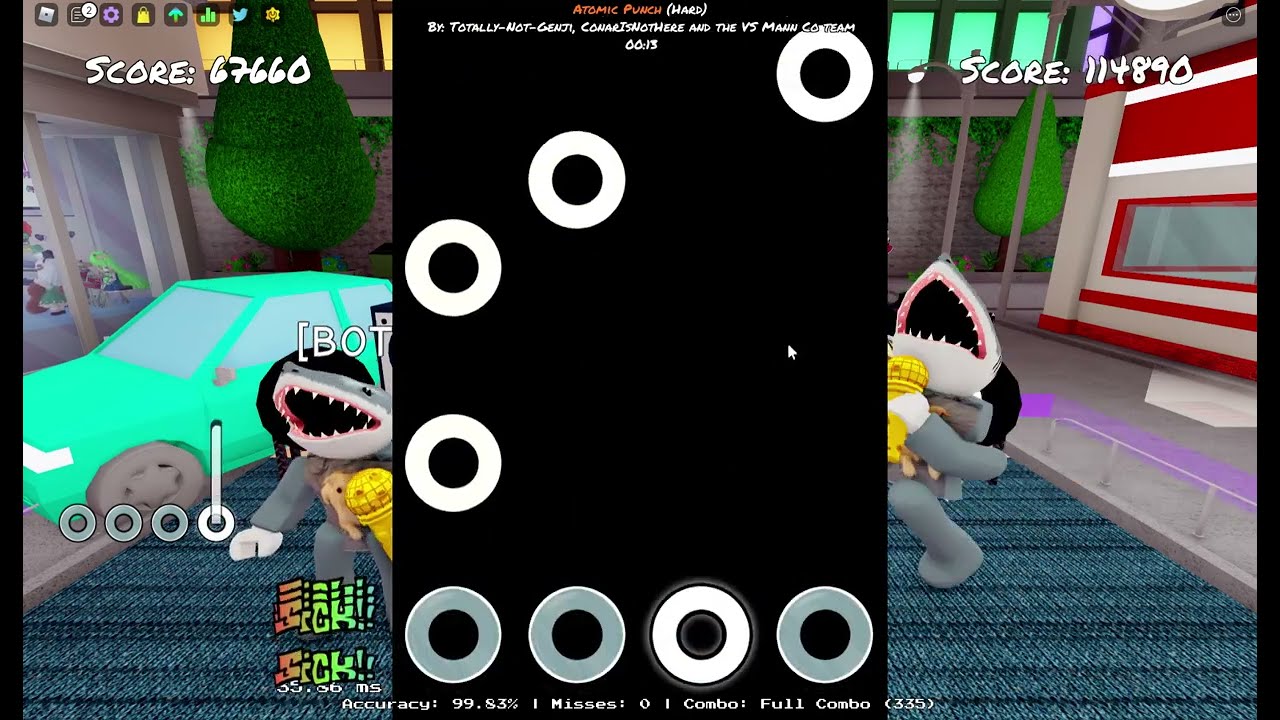The image appears to be a screen capture from a video game, specifically showing two main sections. The central part of the image is dominated by a black vertical rectangle that stretches from the top to the bottom. This black box is peppered with gray and yellow circles, probably indicating game elements or statistics like accuracy, misses, and scores. Notably, the top of this box displays white and orange text, including phrases like "Atomic Punch Hard" and "Totally Not Gentee." There are also numbers at the top corners representing scores, such as "114890" on the top right and "67660" on the top left.

In the background, the scene unveils a room with computer-generated graphics. Two cartoonish sharks are visible, seemingly dancing and holding something yellow, perhaps in shark costumes. The room features a blue carpet in the middle, bordered by gray flooring on either side, and has a distinct red, white, and gray wall on the right side. Also noticeable in the background are two well-manicured, conical trees that resemble pine trees. Additionally, a light teal car is parked on the left side of the scene, contributing to the complex and whimsical environment resembling a playful, indoor setting.